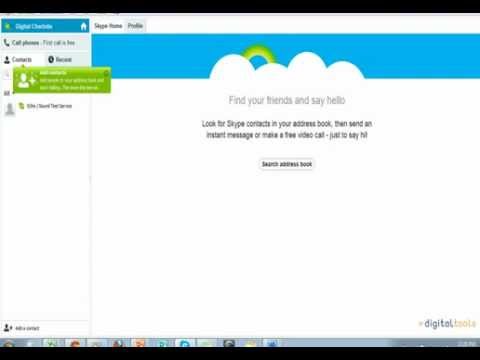This screen capture displays a low-resolution image of a computer desktop with an open application, likely an internet calling app resembling Skype but with an unfamiliar interface. The image quality is notably poor, making specific details challenging to discern. 

At the bottom of the screen, the Windows taskbar is visible, displaying the Start button on the far left alongside several application icons, though they appear indistinct due to partial obstruction by a black bar. Another black bar spans the top of the screen, further contributing to the difficulty in identifying the precise contents.

The primary portion of the screen shows an application window with a predominantly white background, accented with blue and green elements. In the upper left-hand corner, a phone icon is accompanied by the text "Call Phone," and beneath it, a person icon is visible, all situated within the left sidebar.

At the very top of the application window, there seem to be two or three tabs, but their labels are blurred and unreadable. Centrally, the application features a speech bubble icon with the text "Find your friends and say hello," followed by additional smaller text and a clickable button, likely intended for locating and connecting with friends.